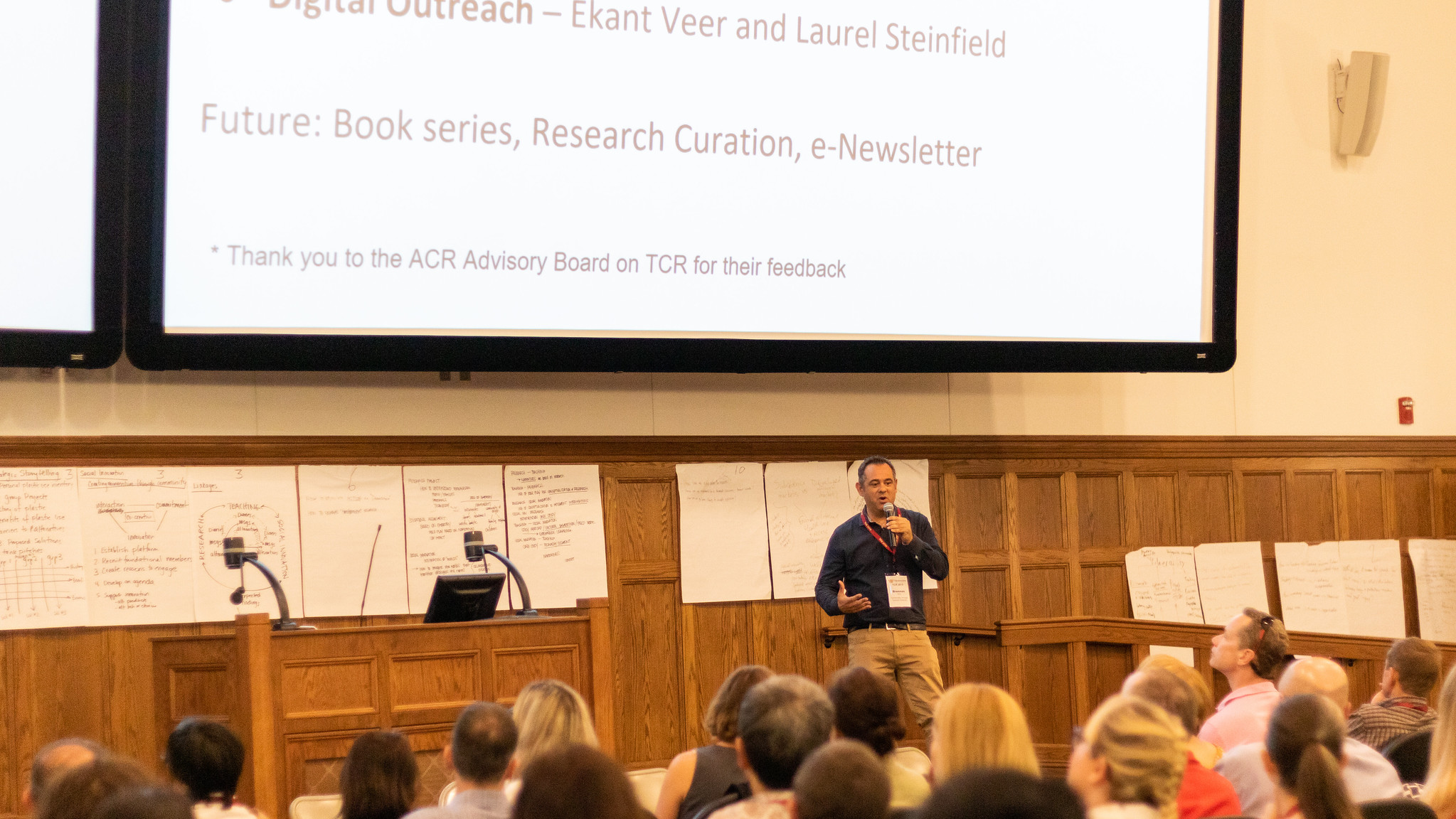In this indoor lecture hall, a well-dressed man stands at a centrally positioned podium, holding a microphone and wearing a red name badge and a card around his neck. He is delivering a speech to a large audience that fills the lower portion of the image. Behind him, several dry erase boards and paper posters adorn the wall, displaying diagrams and phrases. Above his head, a large projected screen prominently features the text "Outreach, Cantvier and Lauren Steinfeld: Future Book Series, Research Curation, E-newsletter.” Additional text on the screen includes a thank-you note to the ACR advisory board on TCR for their feedback. The walls of the room are painted in warm shades of peach or tan with wood paneling, and a fire alarm is visible in the background. The setting is well-lit, suggesting the event is occurring during the day.